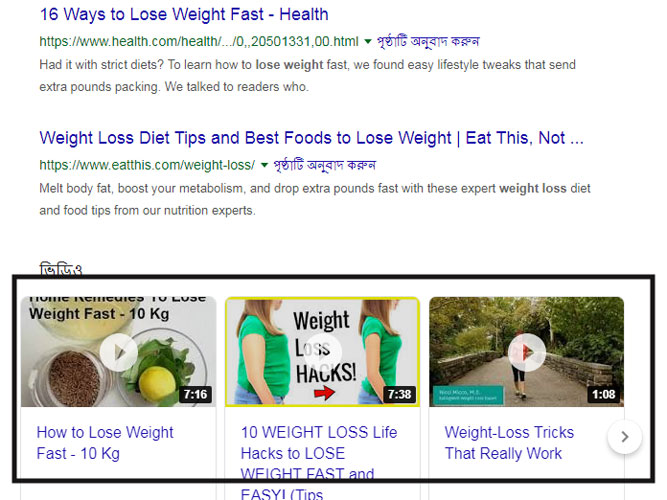A vertical screenshot displays a typical search results page against a plain white background. At the top, the search result's headline appears in blue text: "16 ways to lose weight fast-health." Below that, the web address is shown in green, accompanied by several symbols in another language in blue text.

The main snippet reads in black text: "Had it with strict diets? To learn how to lose weight fast, we found easy lifestyle tweaks that send extra pounds packing. We talked to readers who..." 

Further down, a secondary headline in blue text states: "Weight loss diet tips and best foods to lose weight. Eat this, not..." This is followed again by a green web address and more blue symbols in another language. The accompanying text reads: "Melt body fat, boost your metabolism, and drop extra pounds fast with these expert weight loss diet and food tips from our nutrition experts."

Beneath the text, a long rectangular box with a black border contains three clickable video thumbnails. Each video has a play button at its center:
1. The first video is titled "How to lose weight fast."
2. The middle video is labeled "10 weight loss life hacks to lose weight fast and easy tips."
3. The last video features "Weight loss tricks that really work."